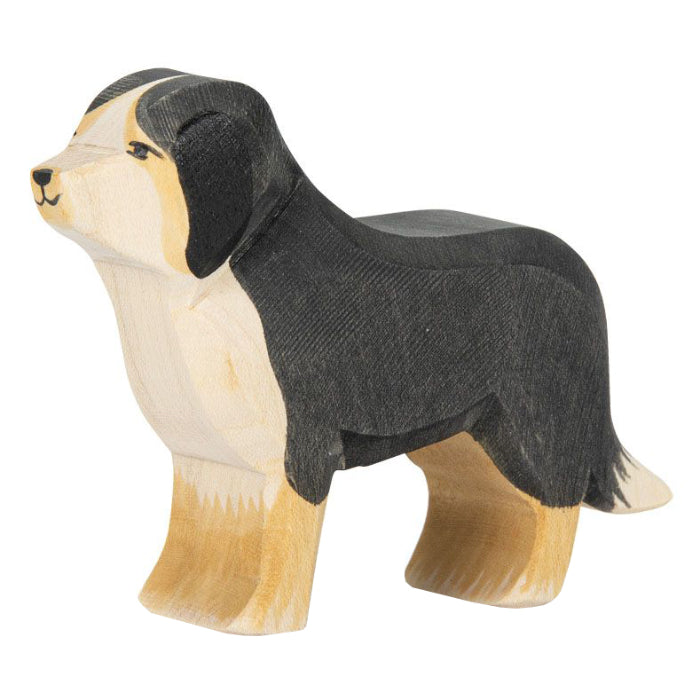This image features a handcrafted wooden sculpture of what appears to be a Burmese mountain dog. Set against a white background, the carving has a roughly hewn, almost childlike quality to it, providing a charming, rustic appeal. The dog's body, while simple and blocky, shows a bit of dimension and has had its hard corners shaved down to softer, more organic shapes. 

The sculpture is painted with a mix of black, tan, and white. The legs are tan, as is the muzzle and the area around the eyes. The back, top of the head, and the base of the tail are black, while the tip of the tail and the chest are white. The eyes, nose, and mouth are very simply painted, consisting of basic dots and lines that evoke a pleasant and content expression.

The front and rear legs of the sculpture are fused together rather than sculpted apart, likely to provide stability and durability. This charming piece, seemingly pulled from its frame and matting for what could be an online advertisement, such as on Etsy, radiates a homemade charm and is sure to take pride of place on someone's shelf. The overall appearance features a pleasant facial expression, giving life to the stylized and endearing representation of the dog.